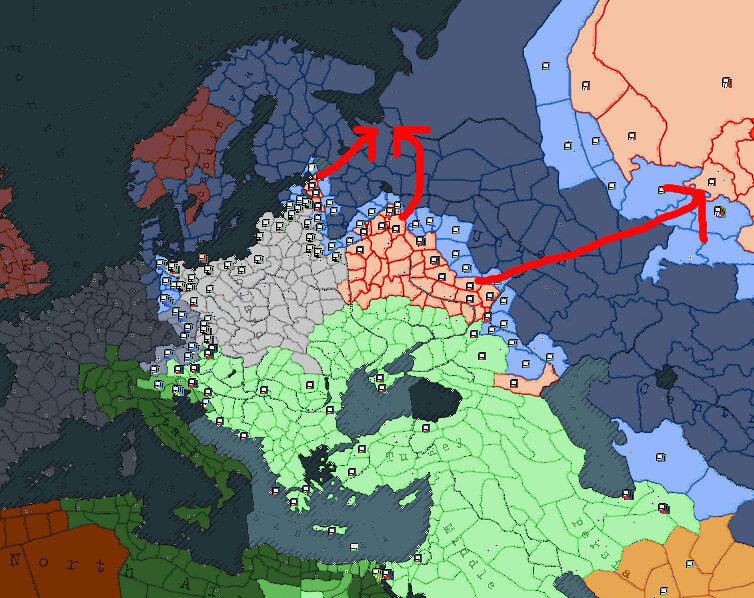The image is a digital, computer-generated map of Europe, easily identifiable by the recognizable shape of countries like Italy, which is depicted in dark green. The map is not a satellite view but rather a color-coded representation, displaying different countries in various shades of blue, peach, green, and red. Italy stands out with its dark green color and is further divided into provinces or states, with boundaries marked in an even darker green. The Mediterranean Sea is displayed in different shades of dark blue surrounding Italy’s boot-like shape. Additional details include numerous lines segmenting each country into smaller sections, possibly indicating counties or states. At the top-center of the map, there are three red arrows, seemingly added via a computer program, with two pointing to one area and another pointing to the right. Scattered across the map are several small square symbols, adding further details to the regions.